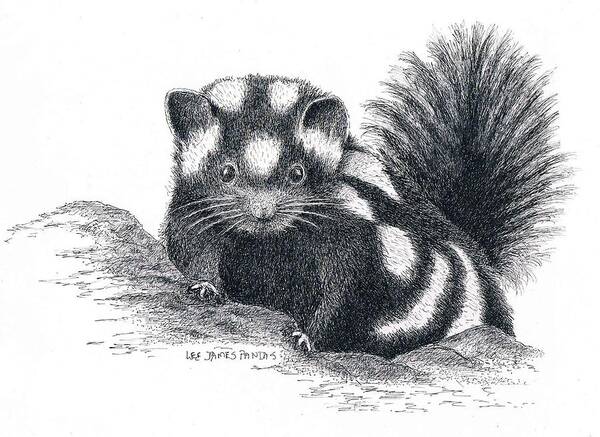This detailed black and white pencil drawing captures a unique animal that bears some resemblance to both a skunk and a squirrel. The creature, depicted with mostly dark fur and white patches scattered over its head and body, stands out vividly against a blank background. It possesses a bushy tail that stands straight up, resembling a pine cone, and its whiskered face looks directly forward. The animal's front paws, each with three toes, rest on a small mound in the landscape, while its back legs remain hidden from view. The artist, Lee James Pandis, has signed the artwork at the bottom, although the signature is somewhat unclear in its entirety. The simplicity of the background, left completely white, emphasizes the finely detailed rendering of the animal and the texture of its fur and tail.